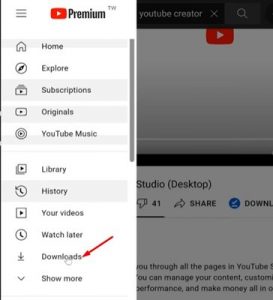Screenshot of a YouTube Premium account interface displayed on a device, possibly a computer or a phone. The screen features a prominent pop-up on the left side, obscuring part of the lighter gray background.

At the top left of the pop-up, there's a white section with the YouTube logo followed by "Premium™". Below it, a menu with three horizontal lines, and underneath that, several navigational icons and labels:
1. A house icon labeled "Home".
2. A compass icon labeled "Explore".
3. An icon labeled "Subscriptions".
4. An icon with an arrow labeled "Originals".
5. A bullseye icon labeled "YouTube Music".
6. An icon with stacked papers labeled "Library".
7. A clock icon with a circular arrow labeled "History".
8. A square icon with a play button labeled "Your videos".
9. A clock icon labeled "Watch later".
10. A download icon labeled "Downloads" with a red arrow pointing to it.
11. A downward-facing arrowhead labeled "Show more".

In the shaded background, partially visible, you can see:
- A search icon.
- The YouTube logo with the text "studio desktop".
- A thumbs-down count showing "41".
- Icons for sharing and downloading.
- Some indistinct text at the very bottom, unclear to the viewer.